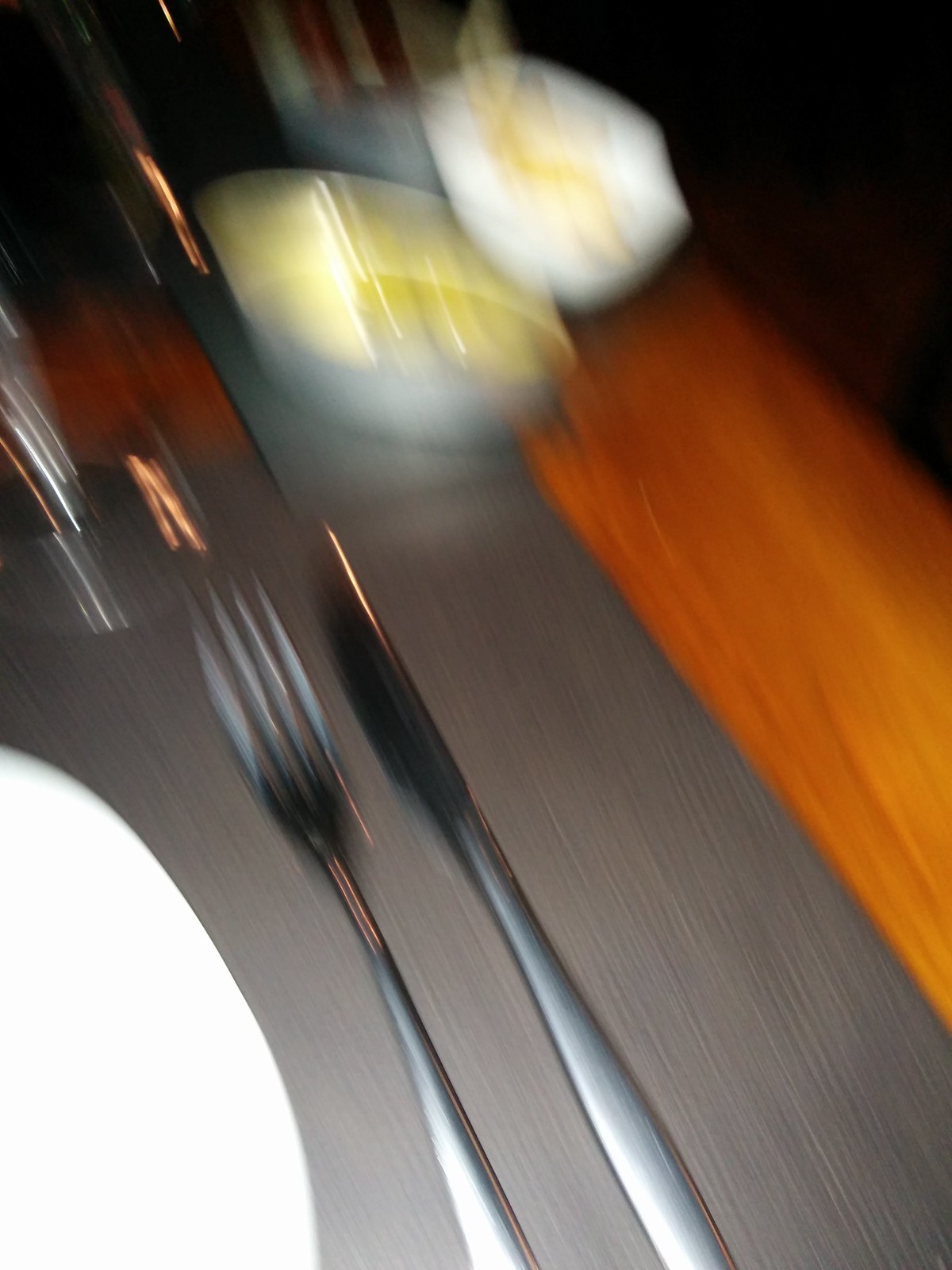This photograph, likely taken accidentally at a restaurant, is extremely blurry and angled, providing a chaotic yet intriguing look at the dining setup. At the center right side of the image, there is a silver napkin on which a fork and knife are laid side by side. The placement of these utensils suggests they are resting on what appears to be a gray placemat. In the bottom left corner, part of a round white plate is visible, hinting at a partially cropped table setting. Toward the top of the photo, there’s an elongated white dish containing a yellow substance, and behind it, a taller white dish filled with ice and an indistinguishable item in the middle. The image's background is predominantly black, creating a stark contrast with the light-colored wooden table’s surface that dominates the composition. The overall blur and stretching of the photograph result in an impression of high-speed capture, further adding to its unintended abstract quality.